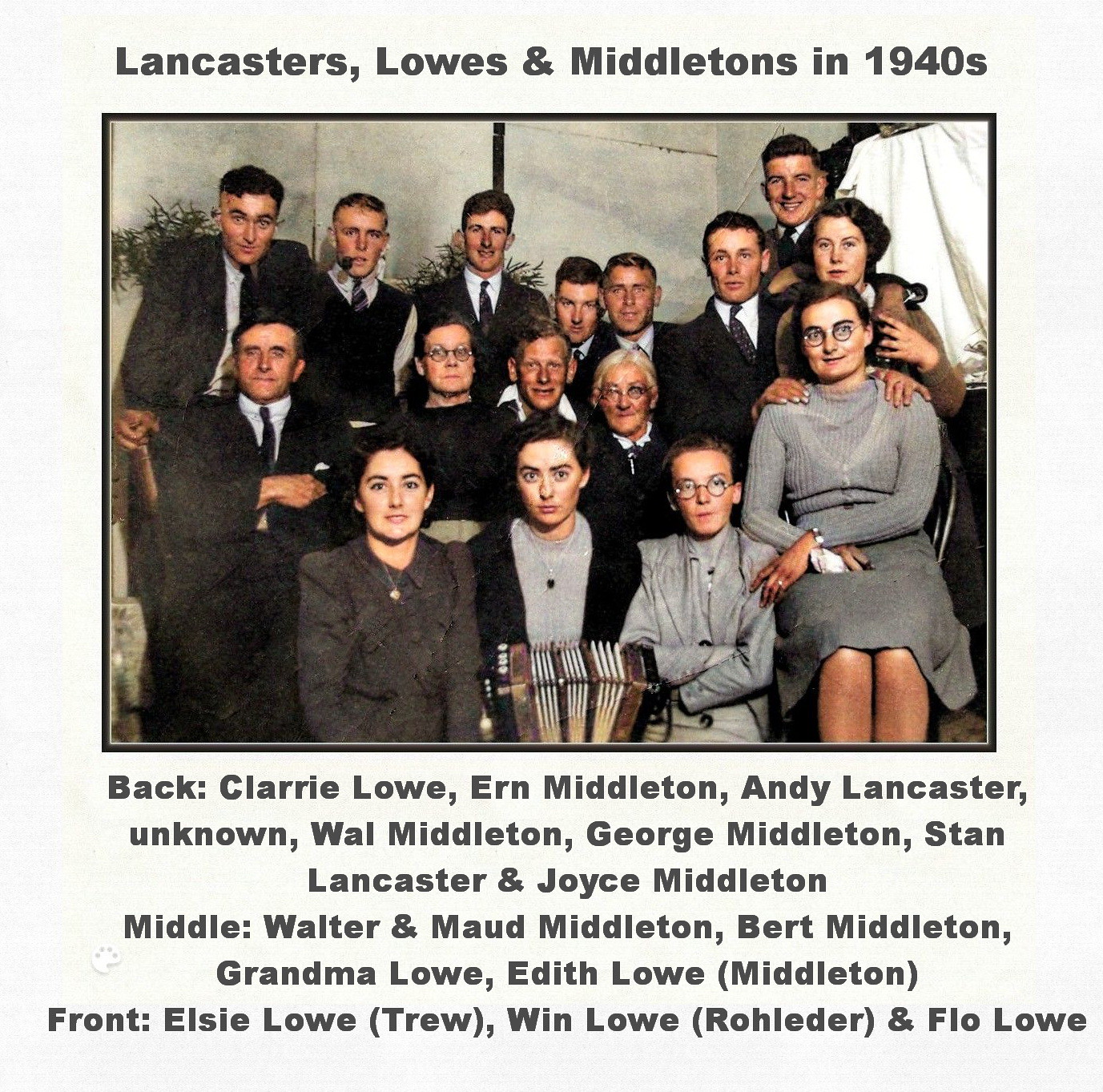This 1940s family portrait, likely from a yearbook or publication, features a large group of approximately 17 individuals, including adults and a few children, all smiling and posing together. The text above the image reads "Lancaster's, Lowe's, and Middleton's in 1940s." Below the photograph, the names of those pictured are listed:

- **Back Row**: Clary Lowe, Ern Middleton, Andy Lancaster, an unknown individual, Wal Middleton, George Middleton, Stan Lancaster, and Joyce Middleton.
- **Next Row**: Walter and Maude Middleton, Bert Middleton, Grandma Lowe, and Edith Lowe Middleton.
- **Middle Row**: Elsie Lowe True, Wynn Lowe, Rod Litter, and Flo Lowe. 

The men are dressed in black suits with ties, while the women wear gray conservative dresses. The backdrop is simple and white, with the photograph framed in black, giving it a timeless and classic appearance.